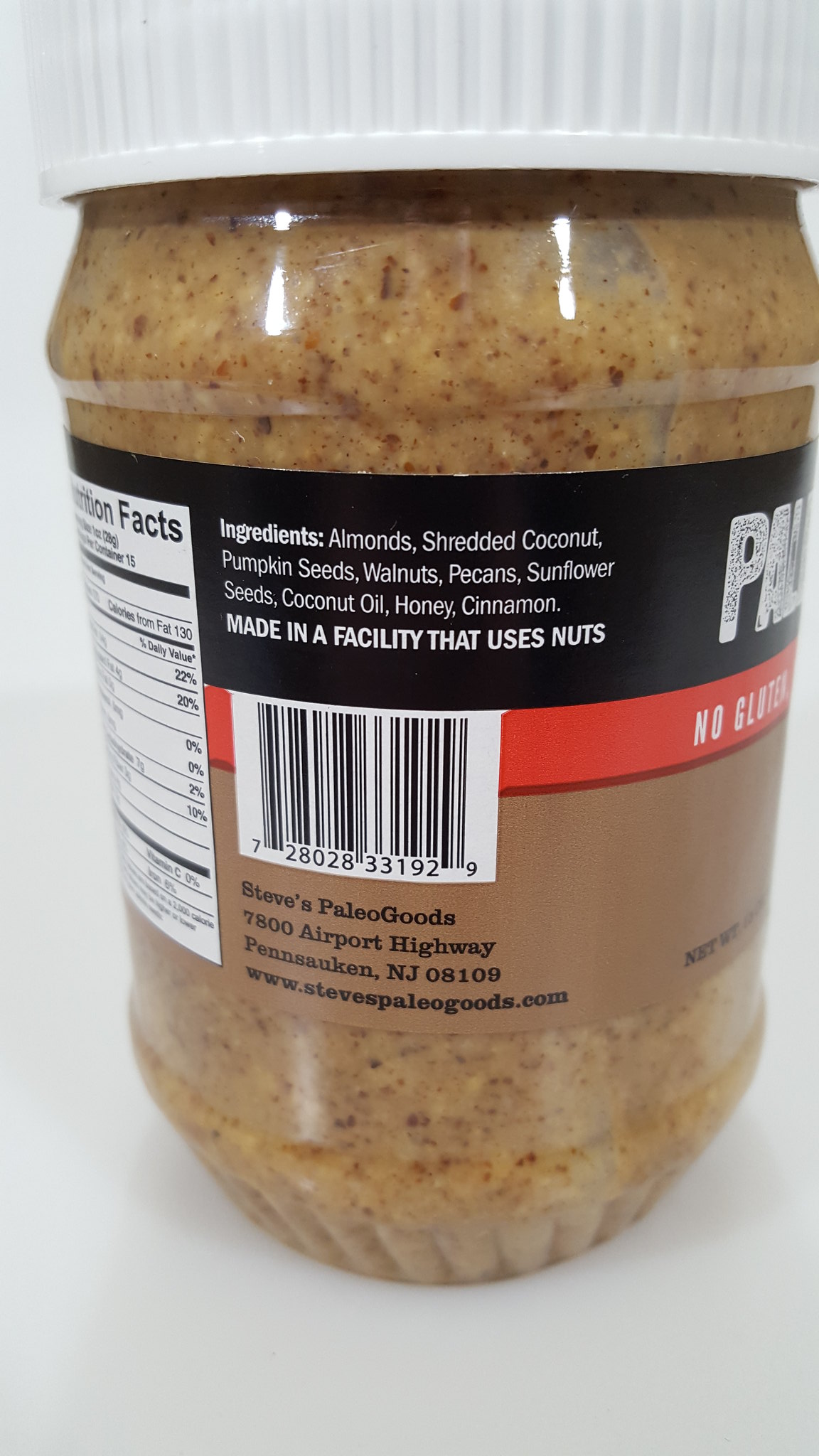This detailed close-up photo showcases a clear, circular plastic jar filled with a brown, speckled mixture, resembling a nut-based butter or paste. The jar has a white, textured, ribbed screw-top lid for better grip. On the left side of the jar, there's a partially visible white square label denoting Nutrition Facts, though only parts of it are legible. The main label, mostly black with an orange and brown band, lists ingredients in white font: almonds, shredded coconut, pumpkin seeds, walnuts, pecans, sunflower seeds, coconut oil, honey, and cinnamon. A red banner underneath states "no gluten." Additionally, the label notes that the product is made in a facility that uses nuts. Prominently featured to the right are bold white letters "PA." Below that is a UPC code "2802833192," and further down on a brown section of the label, it lists the company's address and contact information: Steve's Paleo Goods, 7800 Airport Highway, Pennsauken, NJ 08109, www.stevespaleogoods.com. The background of the photo is grayish, creating a contrast that highlights the jar and its detailed label.